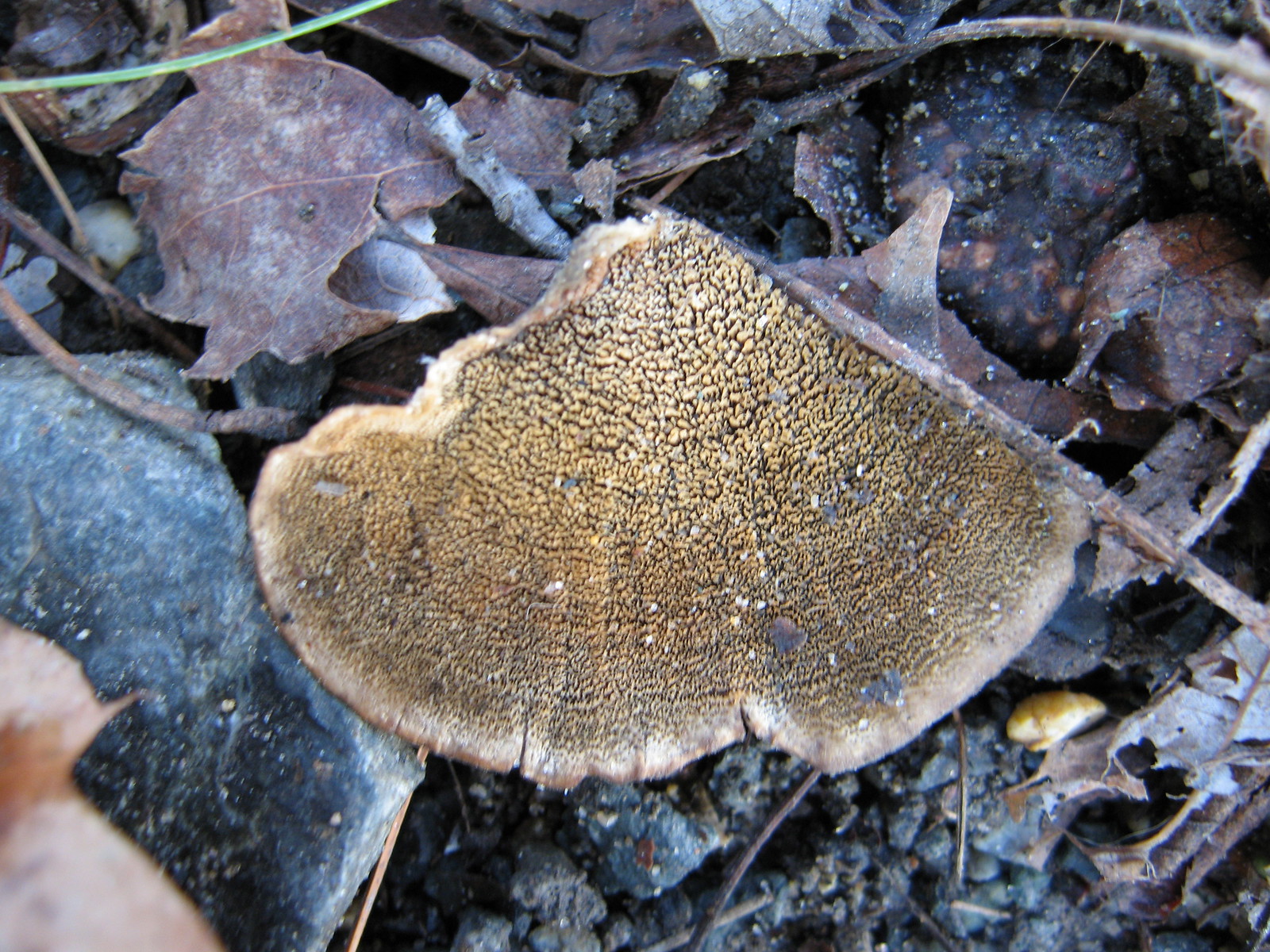In this image, there is a prominent brown and tan object resembling the top of a mushroom, situated outdoors amidst a scatter of twigs, rocks, and a bed of dark brown and gray leaves. The object appears triangular in shape with a quarter-circle curve at its base, featuring a textured surface with curved edges on the left and bottom, and a straight, angled right side. The outer edges of the object have a white tint, enhancing its mushroom-like appearance. It stands out amidst the surrounding decaying, possibly burnt leaves and twigs. A distinct, tan-colored leaf can be seen at the bottom left, providing a contrasting splash of color in the primarily brown and black environment.